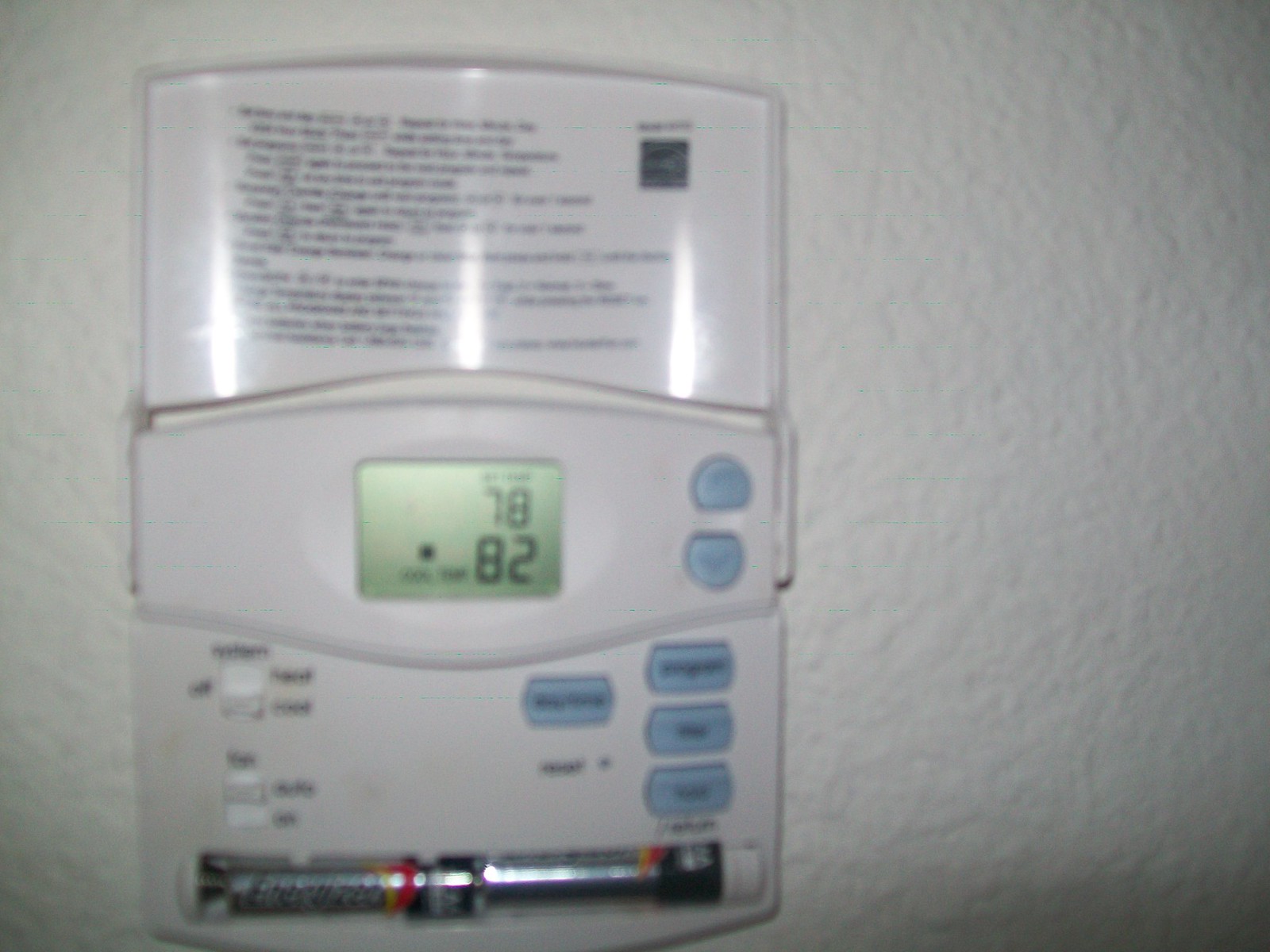This is a close-up image of the controls for a central heating system mounted on a textured white wall, likely wallpaper. The image quality is quite poor, suffering from significant blurriness and overexposure which renders the text on the panel unreadable. The top section of the unit contains a number of instructions, although they are illegible due to the blurriness and excess brightness. Beneath this, a control panel features a green digital display, which distinctly shows the numbers "78" and "82" in a seven-segment format despite the blurriness obscuring other details. The control panel itself is white, accented by two blue buttons below the display. The bottom section includes an additional four blue buttons and two white buttons on either side. Two double AA batteries, silver and black in color, are visibly installed side by side in the unit without a cover, leaving them exposed.